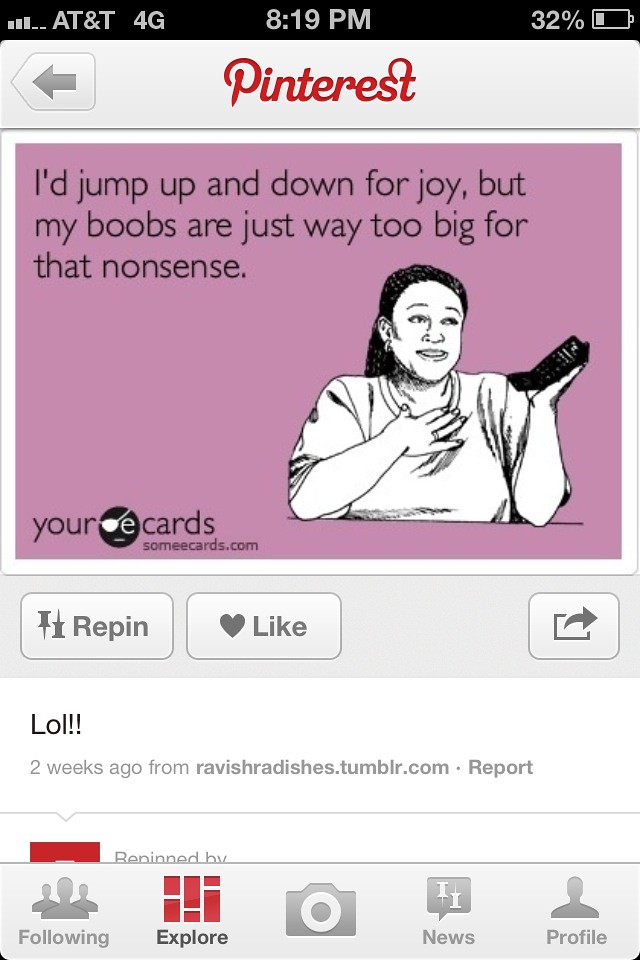This is a detailed description of a meme screenshot taken from Pinterest mobile. The meme features a smiling woman with dark hair, holding a phone in her left hand near her face, and her right hand resting on her chest. The background of the meme is a pinkish-purple hue. The text in black reads, "I jump up and down for joy, but my boobs are just way too big for that nonsense." At the bottom left corner of the image, there is a watermark indicating "Your e-cards, someecards.com."

The screenshot includes the Pinterest interface. The top black bar shows "AT&T 4G," the time "8:19 PM," and the battery level at 32%. Below this, the Pinterest header is visible with a gray bar featuring a back button on the left and "Pinterest" in red font. Directly under the meme image, there are three gray interactive buttons labeled "Repin," "Like," and a share button that looks like a rectangle with a right-pointing arrow. Additionally, below this, there is a comment saying, "LOL!! two weeks ago from Ravish Radishes.Tumblr.com" accompanied by a "report" button.

At the bottom of the Pinterest interface, there are five icons from left to right: a group of silhouettes labeled "following," multiple rectangles labeled "explore," a camera icon, a speech bubble labeled "news," and a silhouette labeled "profile."